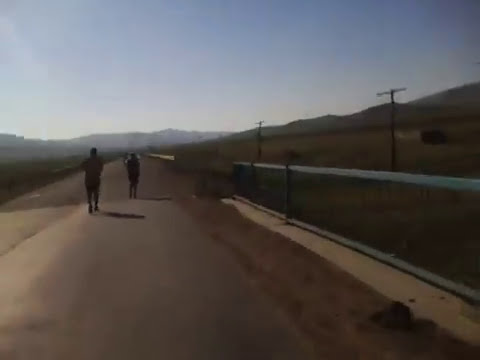The image is a blurry, pixelated square photograph with a slightly shadowy appearance. At the top, an expanse of cloudless blue sky stretches across the frame. Dominating the scene is a road that runs from the bottom left toward the center left, appearing to continue off into the distance. On the left side of the road are two faintly visible figures; one, likely a man, appears to be jogging away from the viewer, while another figure is nearby, possibly walking or also jogging. The right shoulder of the road consists of a dirt area with a blue-colored guardrail spanning from the bottom right to the center right of the image. Scattered telephone poles line this side of the road, progressively fading into the background. The left side of the image features grassland, while the right side eventually opens up to reveal a panoramic view of hills or mountains in the distance. Overall, the scene captures a rural setting with an older-looking road framed by natural landscapes and minimal obstructions.